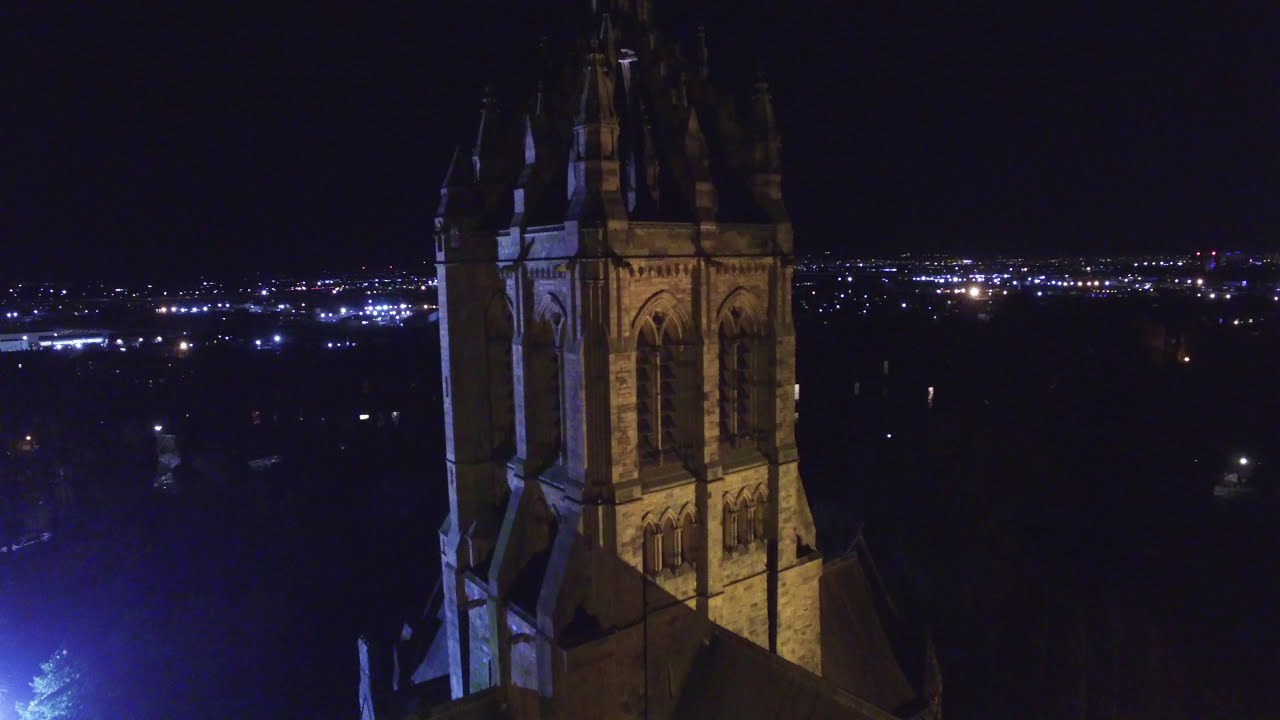This detailed nighttime image, captured in color and landscape orientation, offers an aerial or drone view of a grand, historic tower reminiscent of iconic structures like Big Ben or parts of the Notre Dame Cathedral. The towering stone structure, centered dominantly in the frame, features a multitude of intricate spires and arched openings, exuding a distinctly Victorian, possibly UK-inspired architectural style. The building, appearing tan or grayish in hue, is richly detailed with crests and pointed elements, suggesting an elaborate construction effort. The photograph portrays the top sections of this imposing edifice, likely from the second or third story, viewed from an almost equal height. In the distance, a horizontal line of city lights outlines the horizon against a dark night sky, which consumes the top third of the image. Additionally, there is a faint glow in the water at the bottom left, hinting at ripples or waves, though obscured by the shadows of night. The scene is a striking blend of old-world architecture enveloped in modern urban luminescence.